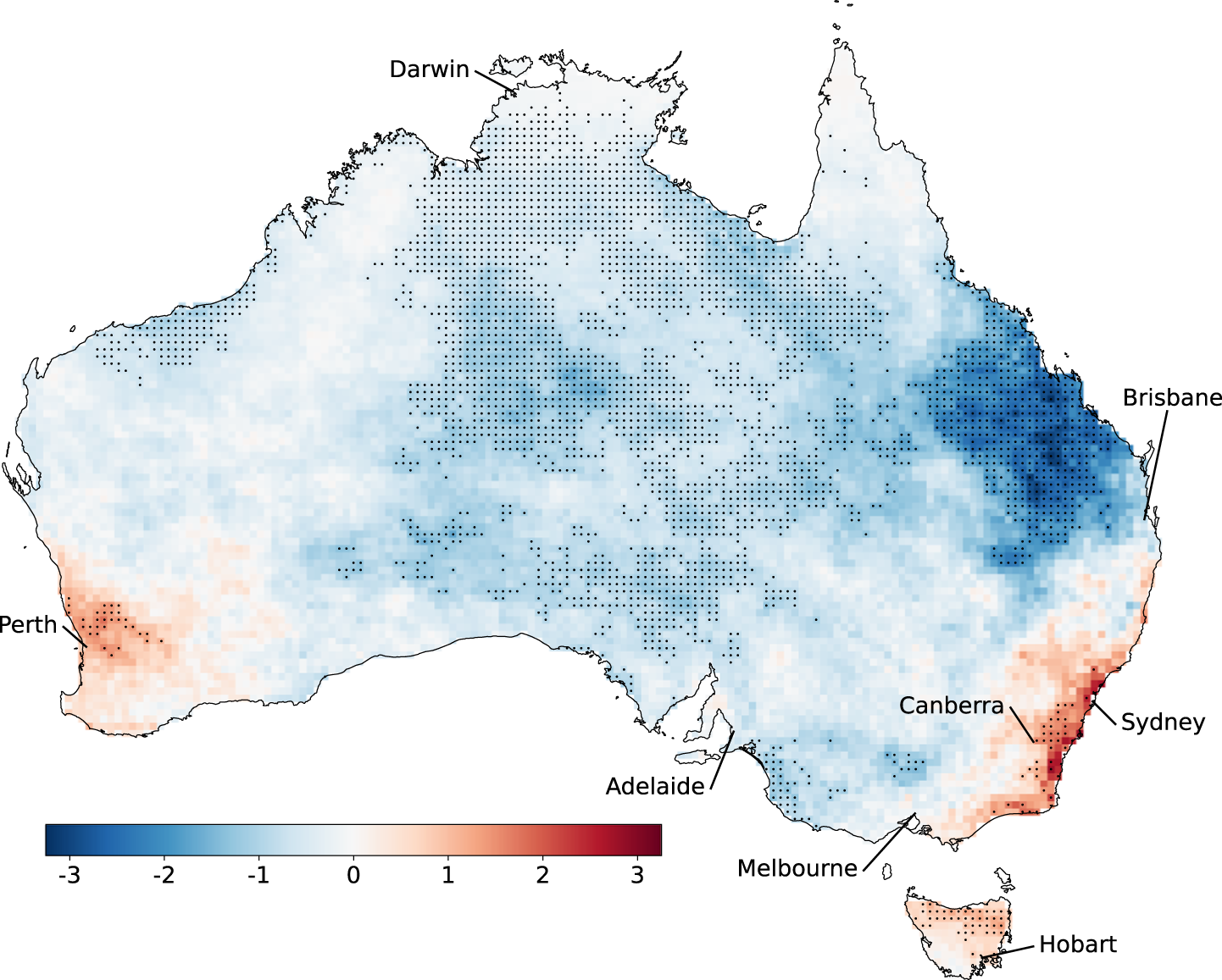This is a detailed, computer-generated map of Australia, distinguished by its thin black outline and vibrant color scheme indicative of a temperature or data gradient. The color scale at the bottom left transitions horizontally from dark blue to light blue, then white, followed by light orange, and culminating in dark red and purple, representing values ranging from negative 3 to 3. The map is densely populated with several labeled cities: Darwin at the top center, Perth on the west coast, Adelaide, and Melbourne towards the south, with Hobart on the nearby island of Tasmania. To the east, it highlights Canberra, Sydney, and Brisbane. The distribution of colors on the map illustrates predominantly blue areas, particularly concentrated in the northwest above Brisbane, indicating lower values. In contrast, red shades dominate around Canberra, Sydney, and Perth, signifying higher values, with the most intense reds near Canberra and Sydney. Scattered across the map are black dots, which are not labeled and do not have a corresponding key, suggesting possibly unknown or less critical data points. The map as a whole appears to convey a heat map-like distribution, with most areas in light blue or white, hinting at moderate values.